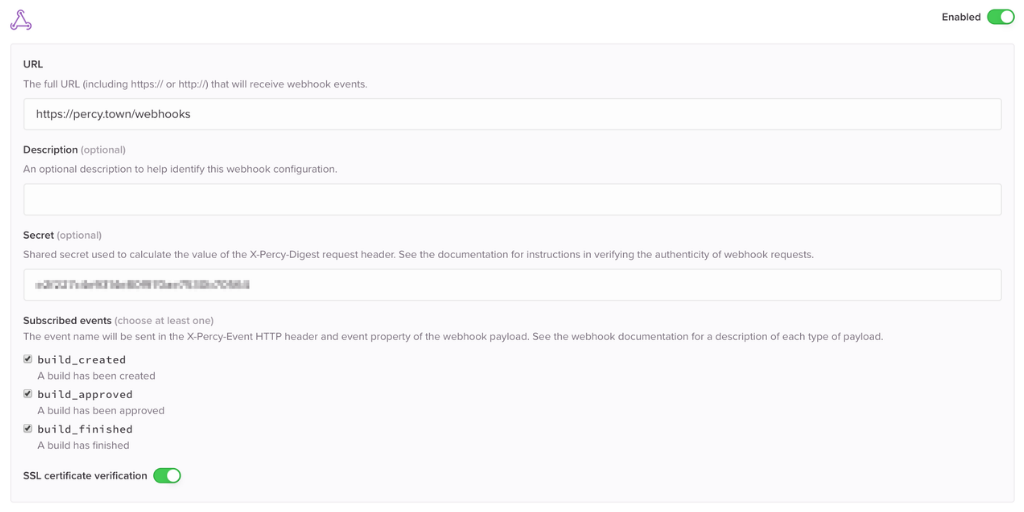Here's the cleaned-up and detailed caption:

"A screenshot of a digital dictionary or encyclopedia page focused on computer coding terminology. In the upper left corner of the screen, there's a triangular icon with rounded corners. On the opposite side at the top, there's a green toggle button labeled 'enabled,' indicating an active feature. The main content is organized with terms followed by concise explanations and examples. The first entry is 'EARL,' explained with a brief description and an example. Below that, the word 'DESCRIPTION' appears in black text, followed by a one-line explanation from a coding perspective. Next is the term 'SECRET,' accompanied by a one-line definition and an example. Further down, 'SUBSCRIBED EVENTS' is detailed with a brief explanation and three examples, each with a checked checkbox. At the end of the page, 'SSL CERTIFICATE VERIFICATION' is listed with an active green toggle switch adjacent to it."